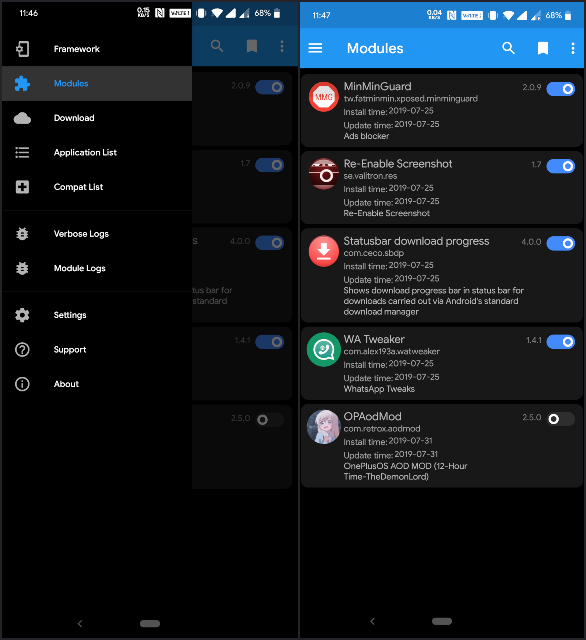This is a detailed screenshot from an unidentified webpage, which is visually divided into two distinct sections. 

The left section features a menu listing various categories: 
- Framework
- Modules
- Download
- Application List
- Compat List
- Verbose Logs
- Module Logs
- Settings
- Support
- About

The right section lists different modules along with specific details for each:
1. **MinMinGuard**
   - **Install Time**: July 25, 2019
   - **Update Time**: July 25, 2019
   - Purpose: Ads Blocker

2. **Re-enable Screenshot**
   - **Install Time**: July 25, 2019
   - **Update Time**: July 25, 2019

3. **Status Bar Download Progress**
   - **Install Time**: July 25, 2019
   - **Update Time**: July 25, 2019
   - Purpose: Displays a download progress bar in the status bar for downloads carried out via Android’s standard download manager

4. **WA Tweaker**
   - **Install Time**: July 25, 2019
   - **Update Time**: July 25, 2019
   - Purpose: WhatsApp Tweaks

5. **OPAODMOD**
   - **Install Time**: July 31, 2019
   - **Update Time**: July 31, 2019
   - Purpose: OnePlusOS AOD (Always On Display) MOD featuring a 12-hour time format called "The Demon Lord"

This structured listing of modules provides detailed installation and update timestamps and outlines specific functionalities, indicating a well-maintained module management interface.